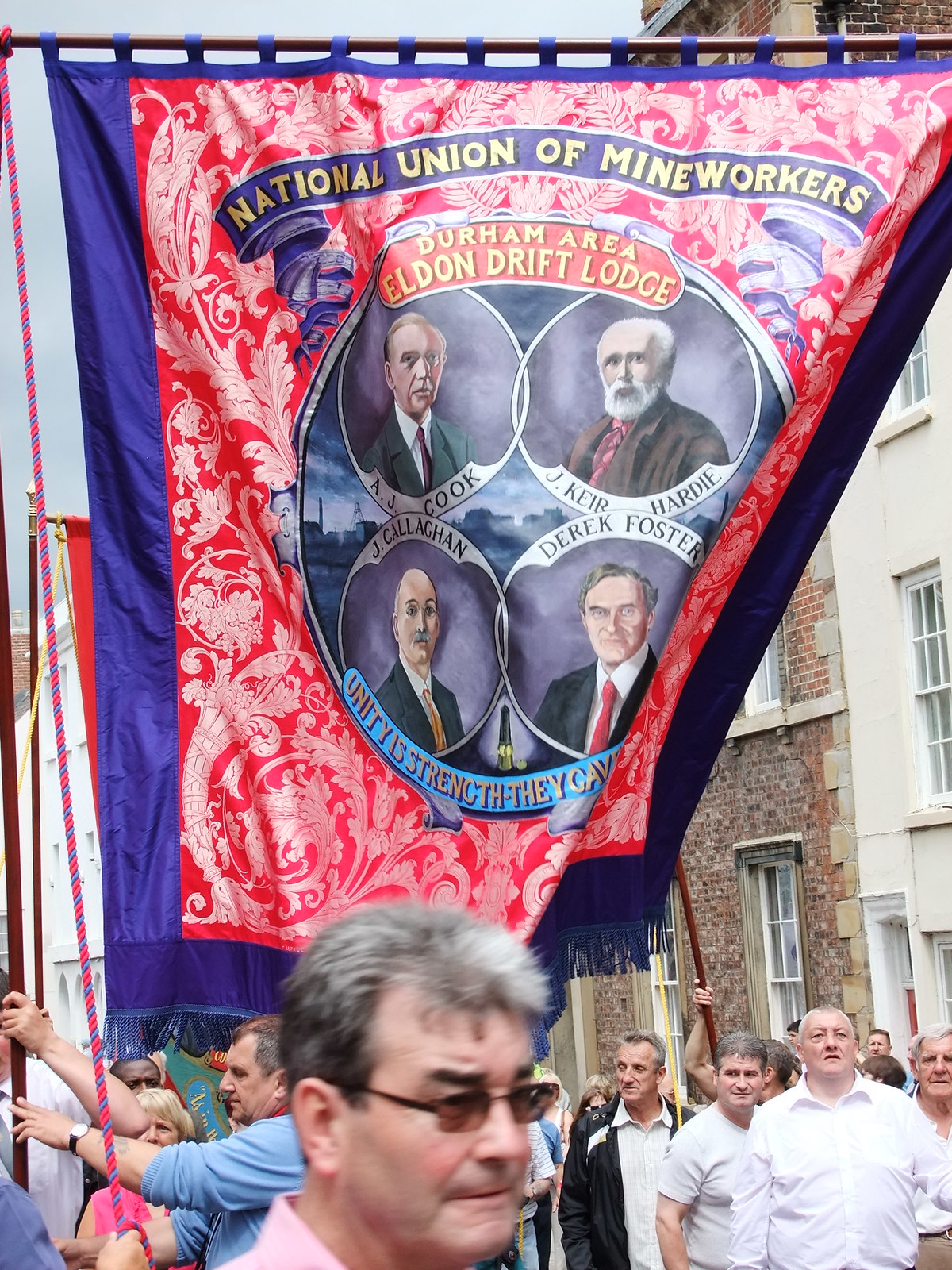The photograph captures a bustling street rally with multiple people, men and women, gathered in support of a cause. Prominently displayed is a large flag held aloft on long, brown poles. The flag is predominantly blue with a decorative frill at the bottom and features a striking red rectangle adorned with intricate silver filigree and floral designs at its center. Within this red section are four painted portraits of men, identified as A.J. Cook, Jay Keerhardy, Jay Callahan, and Derek Foster, with their names captioned either above or below their images. Above these portraits, the words "National Union of Mine Workers" are emblazoned in gold letters on a blue banner, which also includes the text "Durham Area Eldon Drift Lodge." The flag also bears the partially visible slogan "Unity is Strength, They Cave." Surrounding the flag, the crowd is set against the backdrop of a brick multifamily dwelling with white window frames, capturing the unity and diverse participation of this spirited event.